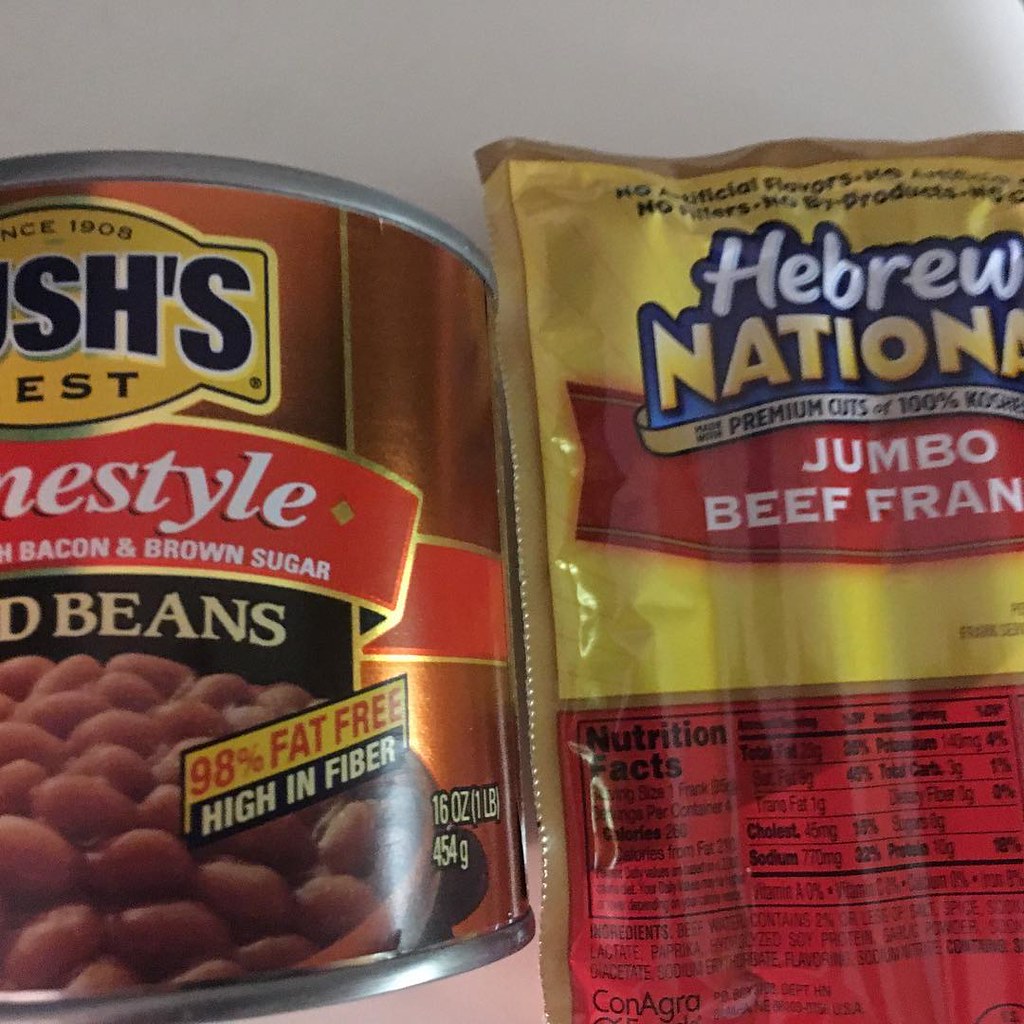This is a detailed, close-up image of two distinct food products side by side on a white background. On the left is a can of Bush's Best Homestyle Beans. The can, with its orangey-copper hue and silver rim, prominently displays a label featuring the words "Bacon and Brown Sugar" in white letters over a red and gold bordered ribbon. The can also highlights that the beans are 98% fat-free and high in fiber, with a photograph of the beans beneath the label. The bottom right corner of the label specifies the weight as 16 ounces (1 LB) and 454 grams.

To the right is a package of Hebrew National Jumbo Beef Franks. The packaging, split into vibrant yellow at the top and rich red at the bottom, features bold, white and yellow text. The label reads "Hebrew National" in large, eye-catching letters with blue shadowing. Beneath it, a navy blue ribbon with a gold trim states "Made from Premium Cuts of 100% Kosher Beef." The red banner at the bottom declares "Jumbo Beef Franks" in bold, white letters, although part of the word "Franks" is cut off. Nutrition facts are printed in black at the bottom of the package.

These products are meticulously described in a vertical rectangular photograph that emphasizes their packaging details and nutritional information.